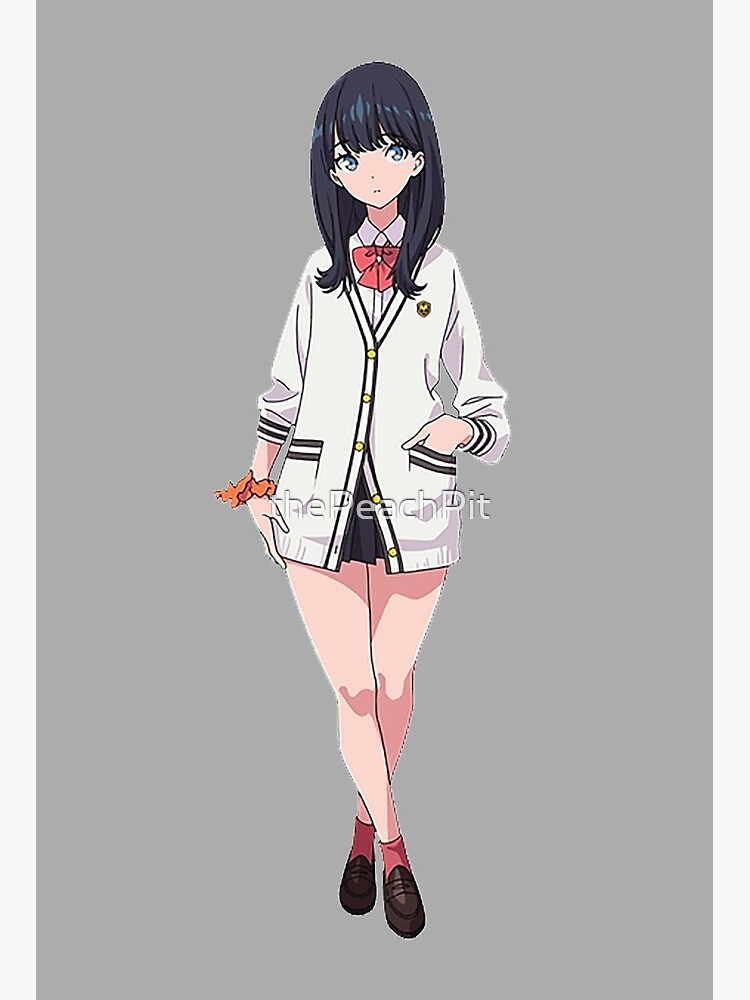This digital anime-style drawing depicts a young woman, either a teenager or a young adult, standing with her legs crossed and facing the viewer against a light gray background. She wears a white cardigan sweater with black trim on the buttons, pockets, and cuffs, which features three yellow buttons fastened in the middle and a hexagonal school logo patch on the upper left side, outlined in gold. Below the cardigan, she sports an extremely short black pleated skirt that reveals her long legs. Her left hand is casually parked in her left pocket, with her right wrist adorned by an orange scrunchie. A red bow tie, reminiscent of a pussy bow, graces the neckline of her white collared dress shirt. Her long, dark hair cascades past her shoulders, complementing her wide, grayish-blue eyes. She completes her look with red ankle socks and dark brown penny loafers. Across the image, in bold letters, is stamped "The Peach Pit."